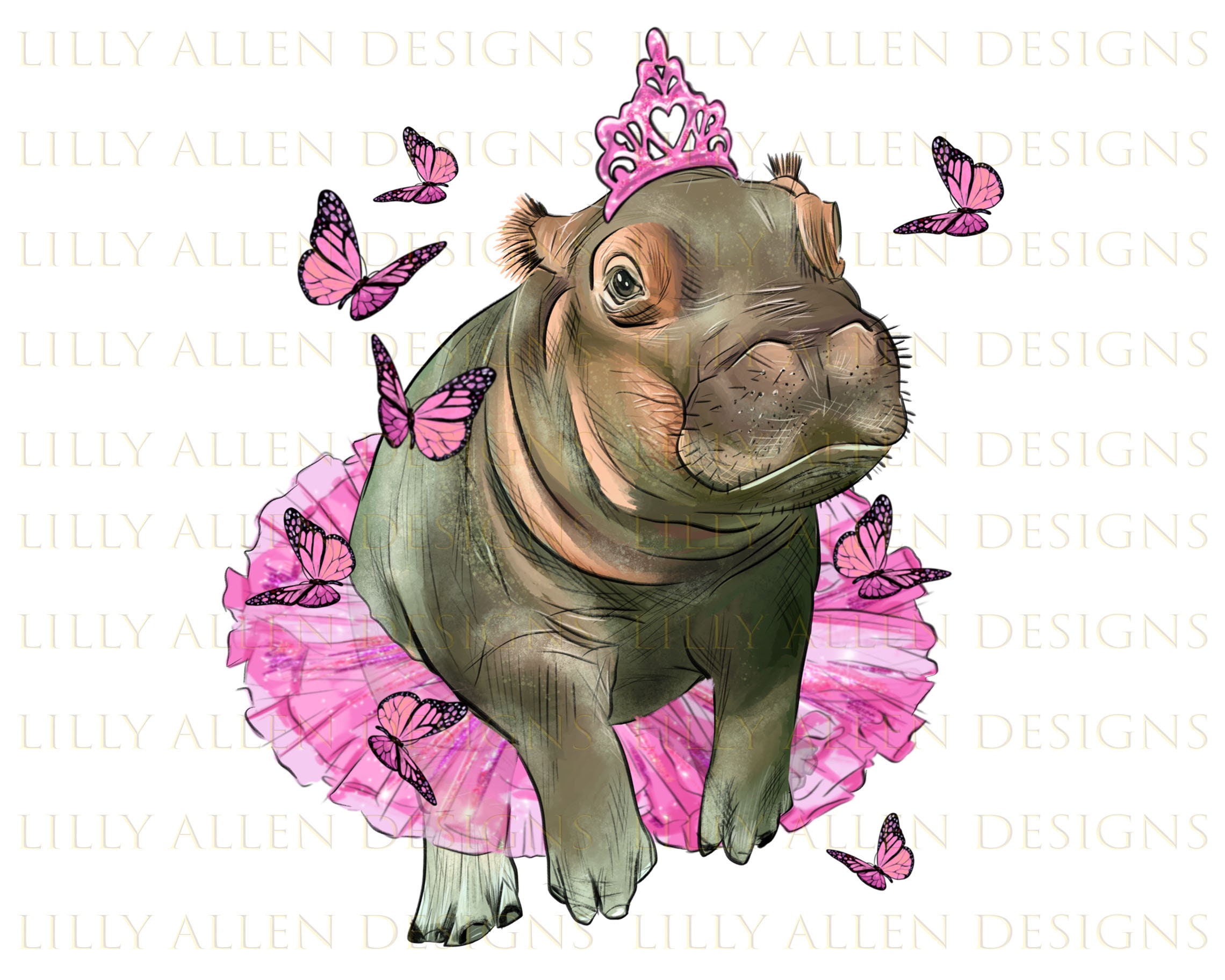The image showcases a detailed illustration by Lily Allen, evident from the watermark "Lily Allen designs" repeated across a plain white background. At the center, a small, gray hippopotamus with dark eyes is depicted standing on its hind legs. The hippopotamus is delicately adorned in a pink ballerina tutu around its waist and a matching pink tiara atop its head. Surrounding the cheerful hippo are eight fluttering butterflies, some pink and black, positioned near its head, around its tutu, and down to its hooves. The animal's skin has visible, lighter fat rolls and coarse hairs around the muzzle, while its neck folds exhibit a pinkish hue, adding texture and charm to this whimsical, ballet-themed drawing.